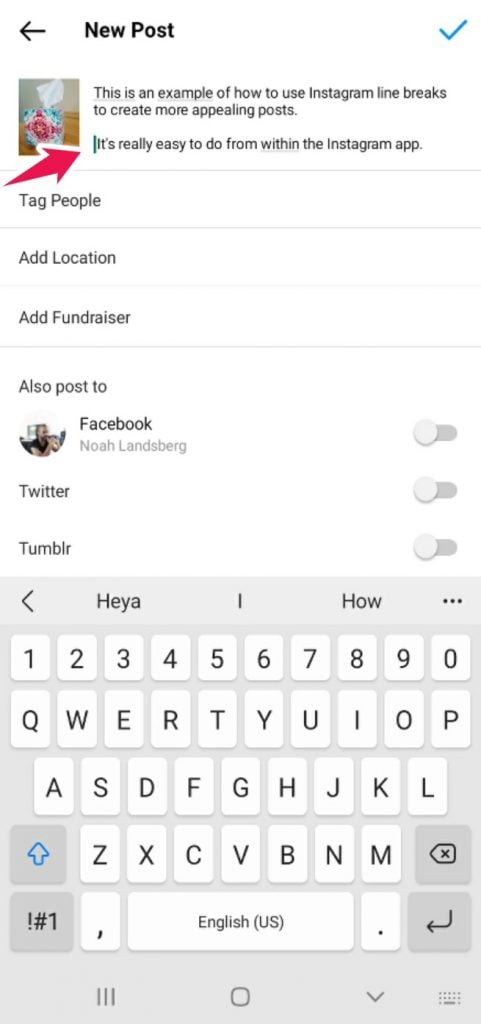This is an image of an Instagram posting interface. At the top of the screen, there's a blue check mark on the right indicating a verified account, and a label that reads "New Post" with an arrow pointing to the left. The image demonstrates how to utilize Instagram line breaks to create more appealing posts. 

Highlighted with a red line and arrow, the photo provides instructions on how easy it is to format posts using the Instagram app. The interface includes several sections: the first section is labeled "Tag People," the second section is "Add Location," and the third section is "Add Fundraiser." 

Below these options, there is a section labeled "Also post to," which allows users to simultaneously share their post on other platforms. This section shows a profile picture of a person named Noah Landsberg. Facebook sharing can be enabled with a toggle switch, currently turned off. Similarly, Twitter and Tumblr toggles are available but are also turned off. 

At the bottom, the standard phone keyboard is visible, with the top row displaying the letters "H E Y a" on the left and "h o w" on the right. Above the '1 2' numbers key, there is a blue arrow pointing upwards, indicating additional keyboard functions. 

This detailed view outlines each element involved in creating and cross-posting an Instagram update.